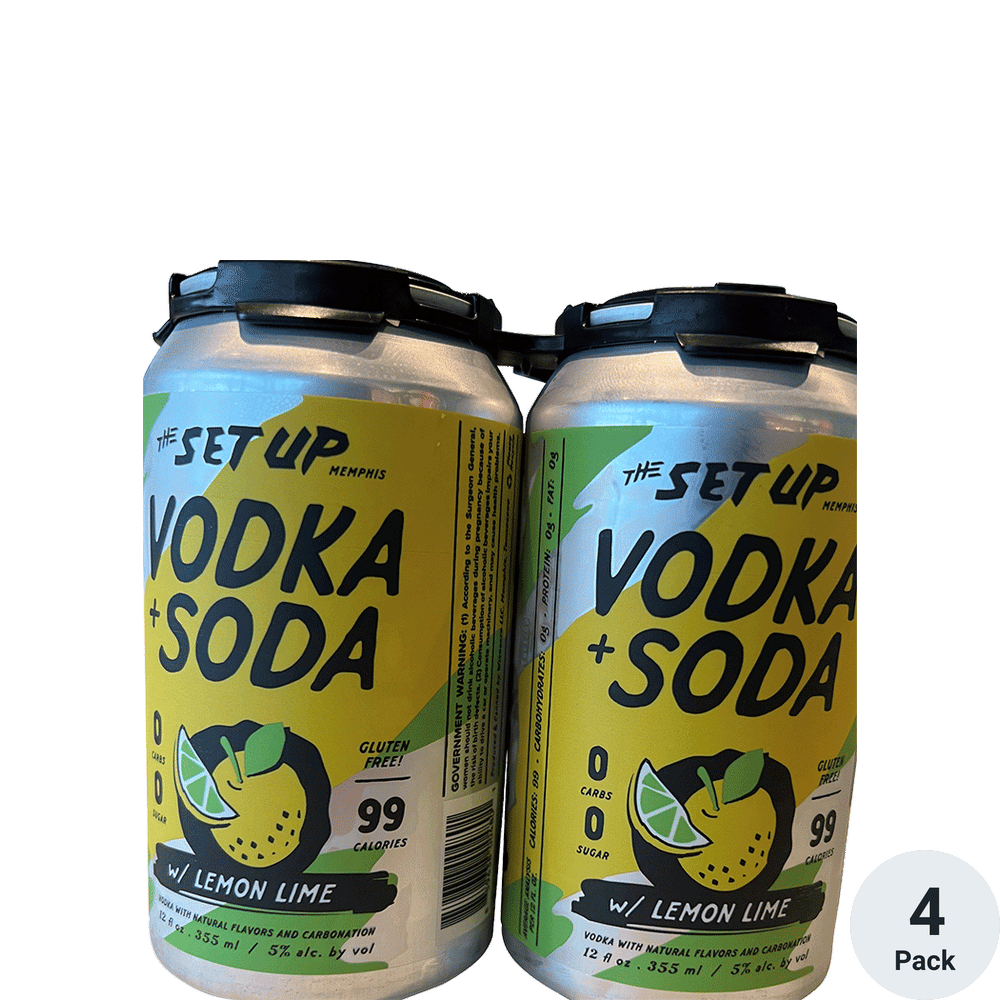This image features an advertisement for Setup Memphis Vodka Soda, a gluten-free canned alcoholic beverage. The focal point shows two silver cans with horizontal yellow and silver stripes, accented by yellow and green designs. Each can is secured at the top with a black plastic connector, though the label indicates it is part of a four-pack. Prominently displayed in black font are the words "Setup Vodka Soda," with nutritional highlights such as "99 calories" and "5% alcohol by volume." Near the bottom of the cans, there is a vibrant depiction of a lemon slice and a lime slice, alongside the text "with lemon lime," which is written in white font on a black background. In the bottom-right corner of the image, a small circular gray area confirms the four-pack packaging.